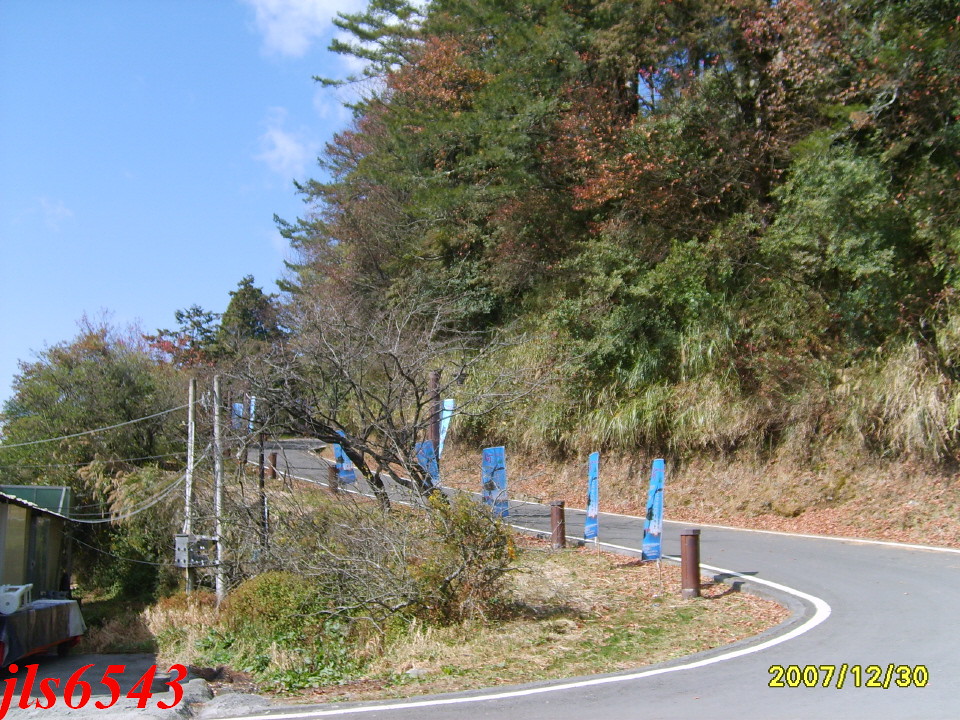The photograph captures a daytime scene along a curvy mountain road that meanders through a rustic landscape. Dry, brown grass and sparse brush dominate the left-hand side, where a stray table sits oddly positioned at the corner amidst strategically placed power lines strung between two short, silver poles. Blue and white cloth banners and colorful temporary signs line the road, resembling perched cones or rolled-up flags. The right side features a mix of large green trees, smaller trees, and one stark, leafless tree, contributing to a varied natural tapestry. A house is partially visible, accompanied by several telephone poles. The road itself is marked by white stripes on both sides, guiding vehicles through its curves. Notably, the scene is time-stamped at the image's bottom right in yellow digits, reading "2007-12-30." Additionally, the lower left corner displays red-lettered text, "JLS6543," adding an extra identifying marker to the photograph.